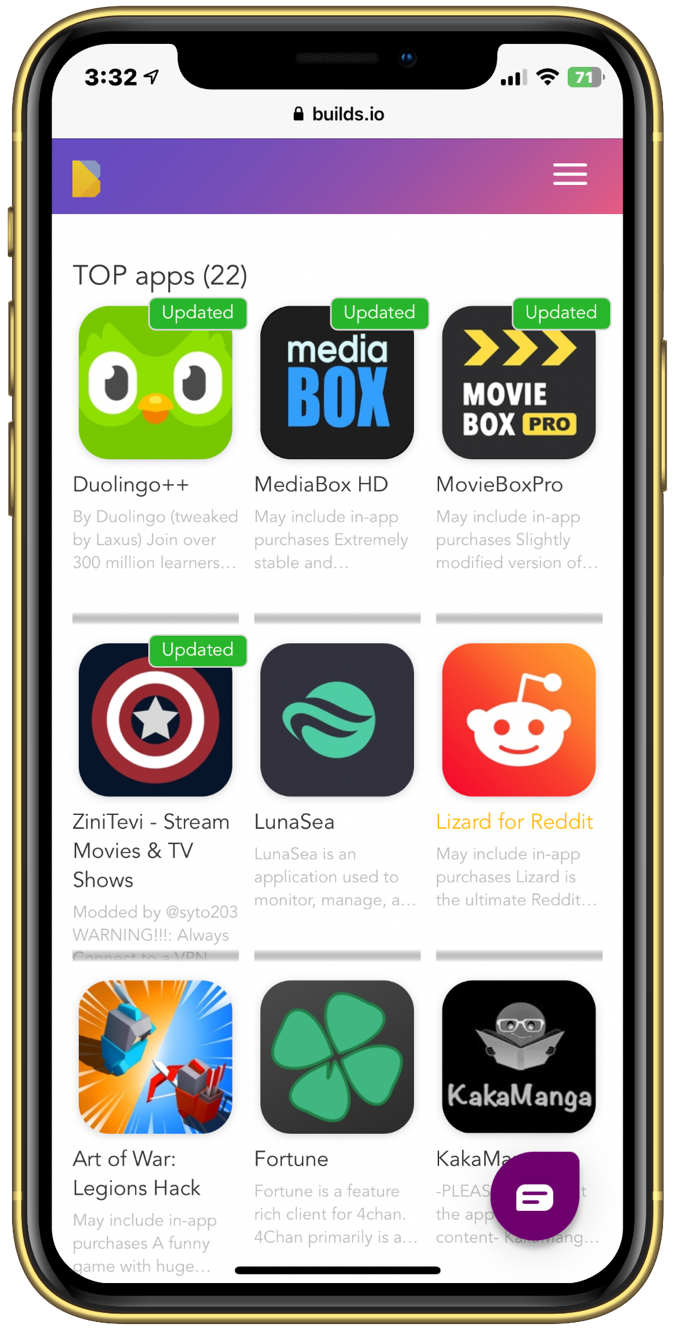The screenshot captures various details from a phone display at 3:32 PM, showing specific elements of the interface:

1. **Status Bar:**
   - **Time:** 3:32 PM
   - **Signal Strength:** 3 out of 4 bars
   - **Wi-Fi:** Connected with full signal
   - **Battery:** 71% Charge

2. **Lock Screen:**
   - **Icon:** Lock symbol indicating that the phone is locked
   - **Website/Service:** Displays "bullds.io" beneath the lock icon

3. **Header Bar:**
   - **Design:** A line that runs from dark purple on the left side to light purple on the right, ending with a hamburger button (menu icon)

4. **Main Content:**
   - **Background:** White
   - **Section Title:** "Top Apps 22"
   - **App Grid:** Organized into three rows with three apps per row. Each app has a small, blurry description underneath that is not legible.
   
   - **First Row:**
     - **Left:** Duolingo
     - **Center:** Double Plus
     - **Right:** MediaBox HD

   - **Second Row:**
     - **Left:** MovieBox Pro
     - **Center:** Zeni Tivi (Stream movies and TV shows)
     - **Right:** Lunacy

   - **Third Row:**
     - **Left:** Lizard (for Reddit)
     - **Center:** Art of War: Legion Hack
     - **Right:** Fortune

   - Note: The exact names and brief descriptions of the apps may vary slightly due to the blurred nature of the text.

This comprehensive elaboration provides an accurate depiction of the screen's contents and the interface layout.